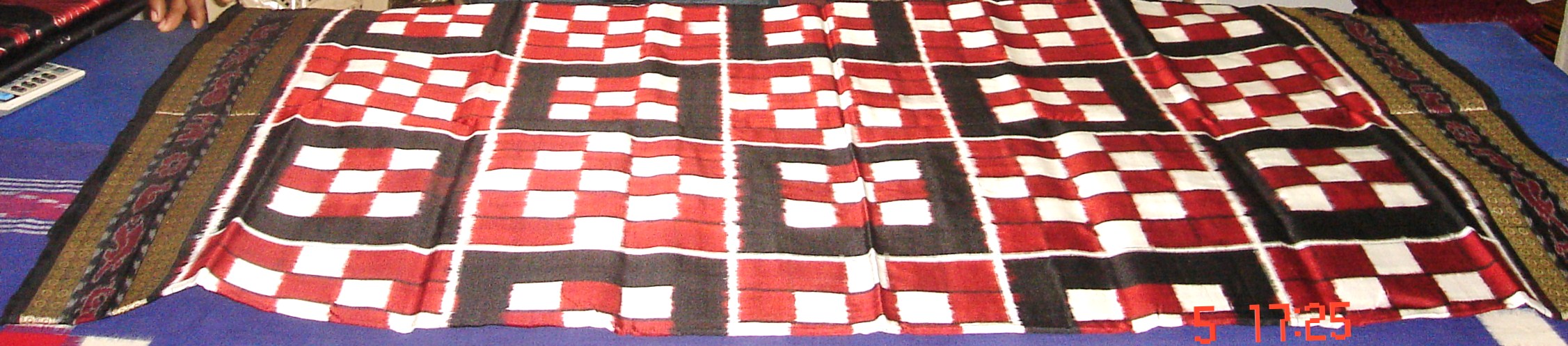The image depicts a large, colorful blanket or bedspread featuring an intricate checkerboard pattern. The central design is composed of squares arranged in five rows of four, each square further divided into smaller red, white, and black checkerboard patterns. The outer perimeter of the blanket is a dark blue, while an inner border features a mix of dark brown, brick-colored, black, and white patterns. A gold fringe with a floral design, showcasing thin red and blue flowers, adorns the edges. Notable is a set of numbers, "5-17-25," located at the bottom, though their significance remains unclear. The overall composition is detailed and complex, with multiple layers of patterns and colors blending harmoniously.